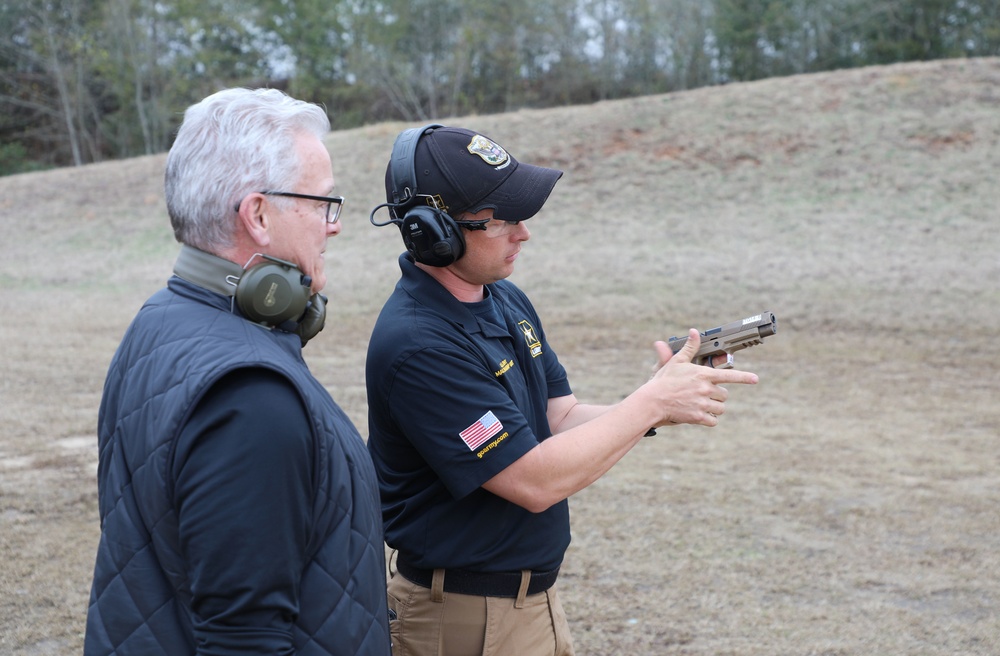In the photograph, two men are positioned facing the right against a backdrop of rolling hills and dense trees with patches of blue sky visible. The man in the foreground, who appears to be a firearms instructor, holds a light brown automatic pistol pointed upwards and to the left. He is wearing a short-sleeved navy blue shirt adorned with an American flag logo on the sleeve, yellow embroidery, and a yellow star on a black background on the right side. His attire also includes tan pants, a dark blue cap, black earmuffs, and protective goggles. His right hand grips the pistol with his thumb up and index finger pointing straight to the left, situated directly under the trigger guard. 

Behind him stands an older gentleman, likely in his 60s or 70s, with white hair and black glasses. He wears a blue vest over a blue long-sleeved shirt, with his green ear guards hanging down over the back of his neck. The older man seems to be receiving instructions, possibly on how to handle the firearm. The background appears wintery with dry grass underfoot and thick green forest in the distance. The entire scene is captured in landscape orientation, placing the focus on the interaction between the two men amidst a serene outdoor setting.